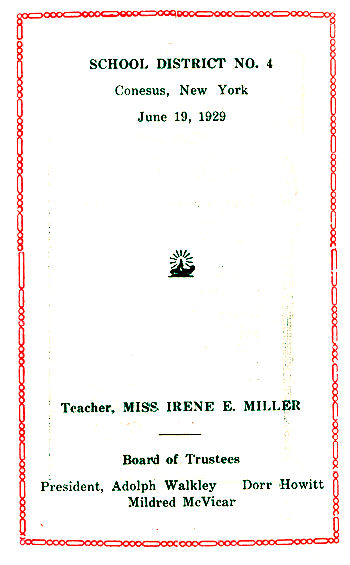The image depicts a vintage pamphlet or announcement from School District No. 4, dated June 19, 1929, in Canisius, New York. The pamphlet has a distinctive border featuring a red dash-dot-dot pattern and some etched designs. The text is primarily in green and includes the school's name and date prominently at the top. Below this, there is a central, somewhat indistinct logo or symbol. Toward the bottom, the pamphlet lists key personnel: the teacher, Ms. Irene E. Miller, and the Board of Trustees members, President Adolf Walkley, Dor Howitt, and Mildred McVicar. The cover shows signs of age with various marks on both the left and right sides.